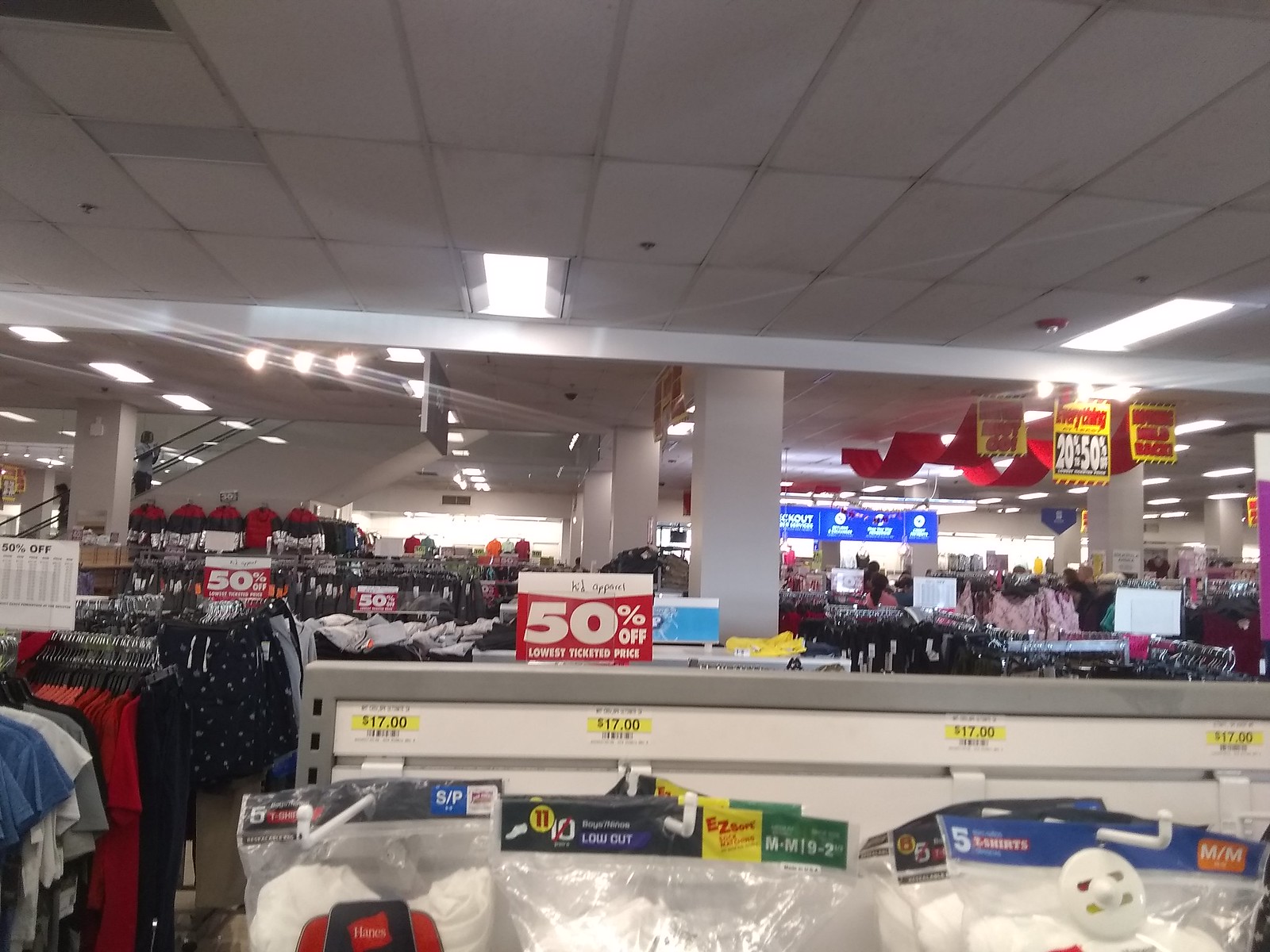This photo captures the interior of a bustling retail clothing store, brightly lit by fluorescent lights mounted on a white tiled ceiling. The scene is defined by a row of white support beams extending from floor to ceiling, creating a rhythmic pattern that leads the eye to a window in the back of the store. Sunlight pours in through this window, illuminating the space. The store is filled with various clothing racks arranged in orderly aisles, showcasing an array of shirts, blouses, and other garments for men and women.

In the immediate foreground, there is a prominent white rack with a gray border, topped by a striking red sign that reads "50% off" in large white letters, drawing significant attention. Hanging on this rack are clear plastic bags containing what appears to be socks or underwear, some marked with a $17 price tag, hinting at a package deal. The background reveals even more discount signs, with offers ranging from 20% to 50% off, scattered throughout the store. The overall atmosphere is busy yet orderly, providing a glimpse into a typical shopping day in a department store.